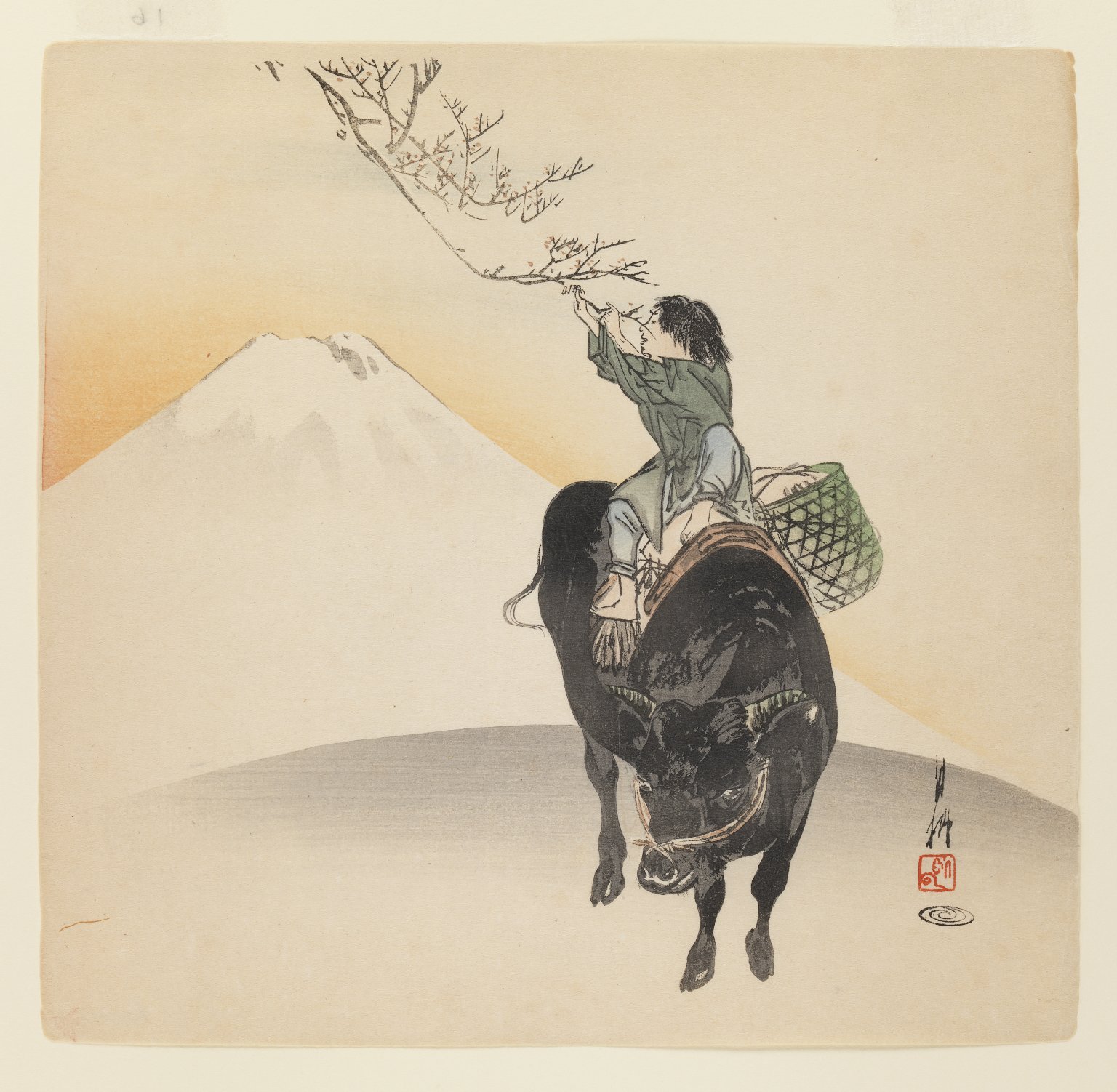This is a vintage, Asian-inspired illustration, possibly a watercolor painting on paper, depicting a scene of a person riding a black ox. The person, who appears to be of Oriental descent, is dressed in olive drab clothing consisting of a shirt and pants. They are barefoot, with black hair. Seated on a blanket or saddle draped over the ox, the person is gathering berries from a branch hanging down from the top of the illustration. Attached to the saddle is a basket, likely used to collect the berries.

The ox, facing the viewer, is entirely black, including its hooves, face, and short horns. The scene is minimalistic, featuring a rusty grayish background with a tall mountain, possibly resembling the Goji Mountain, towering in the distance, adding a sense of depth. On the right-hand side of the illustration, there is Japanese text, enhancing the cultural authenticity of the artwork.